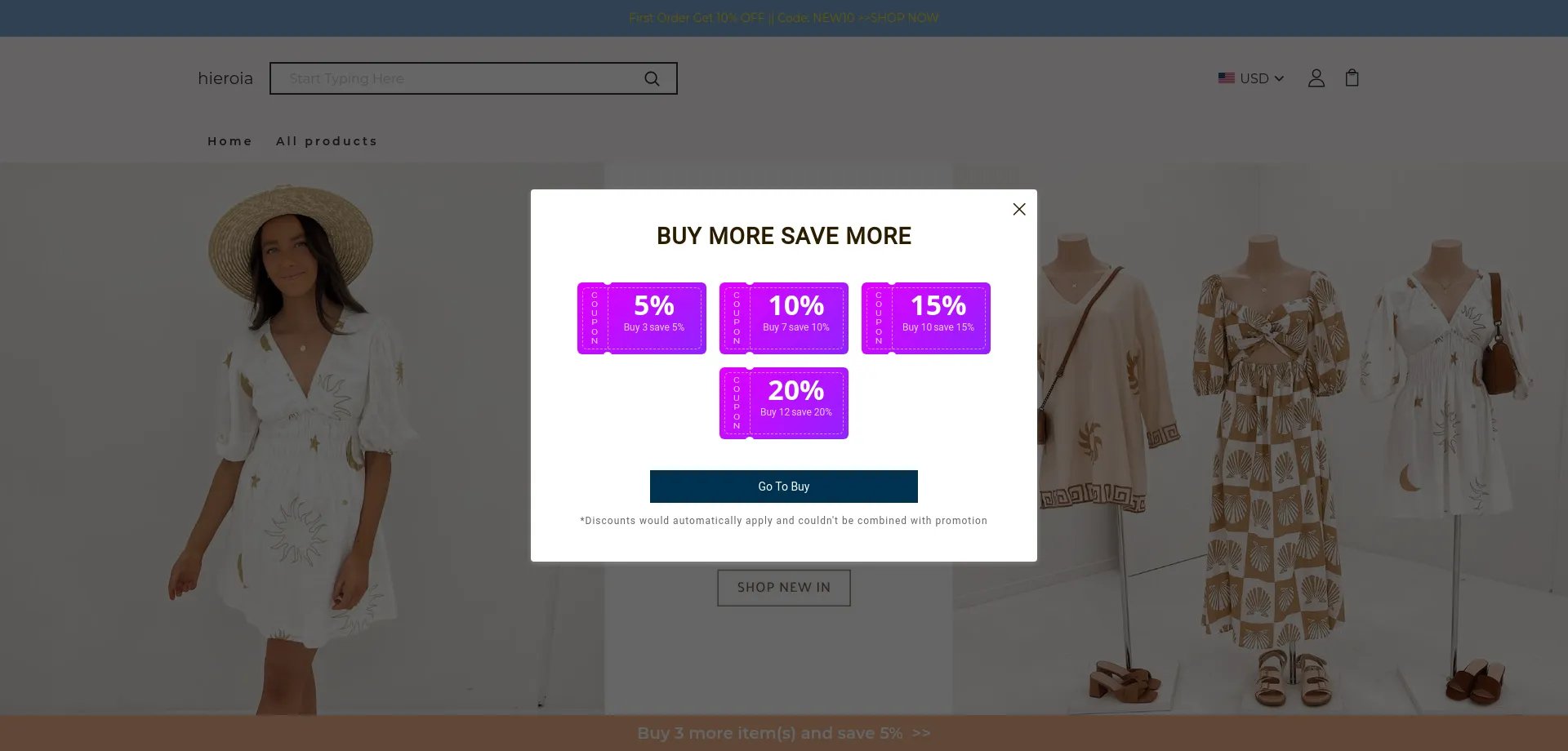This description appears to be of a promotional pop-up advertisement on a clothing website's homepage. Here's a cleaned-up and detailed caption:

---

On the homepage of the clothing website HIEROLA, a bright white promotional pop-up takes center stage against a dimmed background. The pop-up, titled "Buy More, Save More," features four gradient purple tickets, each displaying different discount percentages in bold white font: 5%, 10%, 15%, and 20%. Below the tickets, a blue rectangle with "GO TO BUY" written in white invites users to shop. A note in black font beneath the button explains that discounts will automatically apply and cannot be combined with other promotions. In the background, a woman with dark brown hair and a darker skin tone models a white dress and a wide-brimmed straw hat. Surrounding her are various neutral-toned clothing items, including dresses in tan and cream, a t-shirt with checkered hems, a tan and white square-patterned dress, and a white top featuring silver and gold moon designs. At the top of the webpage, the store's name, HIEROLA, is displayed alongside a search bar with the placeholder text "Start typing here."